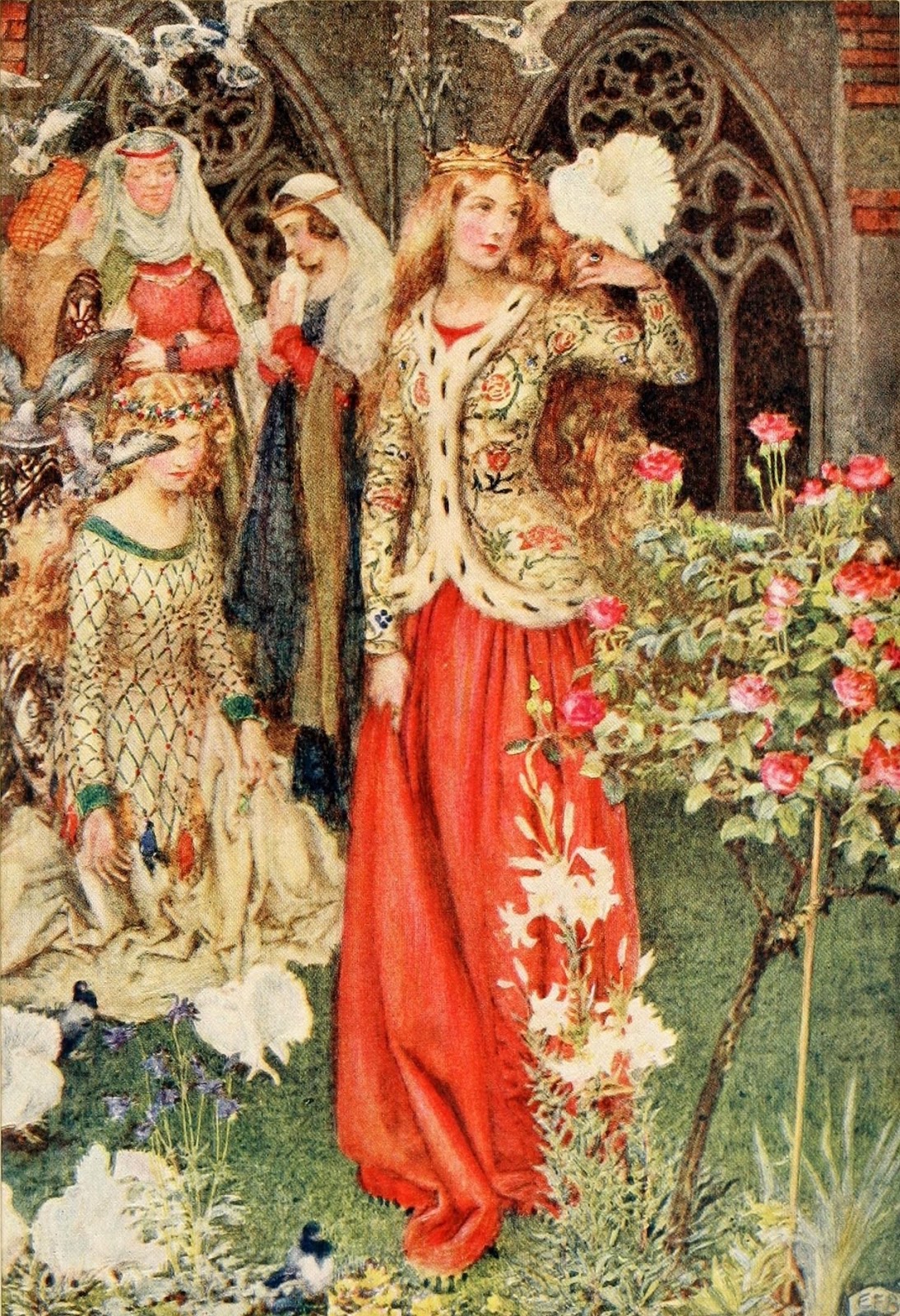In an Elizabethan-style painting set in a courtyard, a young woman stands prominently at the center. She wears an orange-bottomed dress with a yellow, ornate coat adorned with floral and vine designs. The coat has a long fur trim with black lines that cascades around her neck, chest, and waist. Her long, red hair reaches below her waist, crowned with a golden headpiece. She holds her right hand nearly vertical to her body, pointing towards her head, where a white bird perches, capturing her gaze.

To her left, a younger girl crouches on the ground in a yellow dress with green lines and a white bird at the hem of her dress. Behind them, three women stand in a semi-circle: one in a blue dress with a white headscarf bent over a white bird in her hands, another in a red dress with gray hair and arms crossed, wearing a silver crown and a white headdress, and the last with a plaid handkerchief, an amber-sleeved brown vest, and a white and gray bird perched on her head.

A rosebush with a thin brown trunk and small green leaves dotted with roses emerges to the right side. Above the figures, several white and gray birds can be seen flying. The backdrop of the painting reveals what appears to be the front of a church, characterized by dark brown and light brown hues with hints of red brick. Richly colored in greens, reds, blues, and oranges, the scene is filled with grass, flowers, and vibrant Elizabethan attire, evoking an older, timeless ambiance.